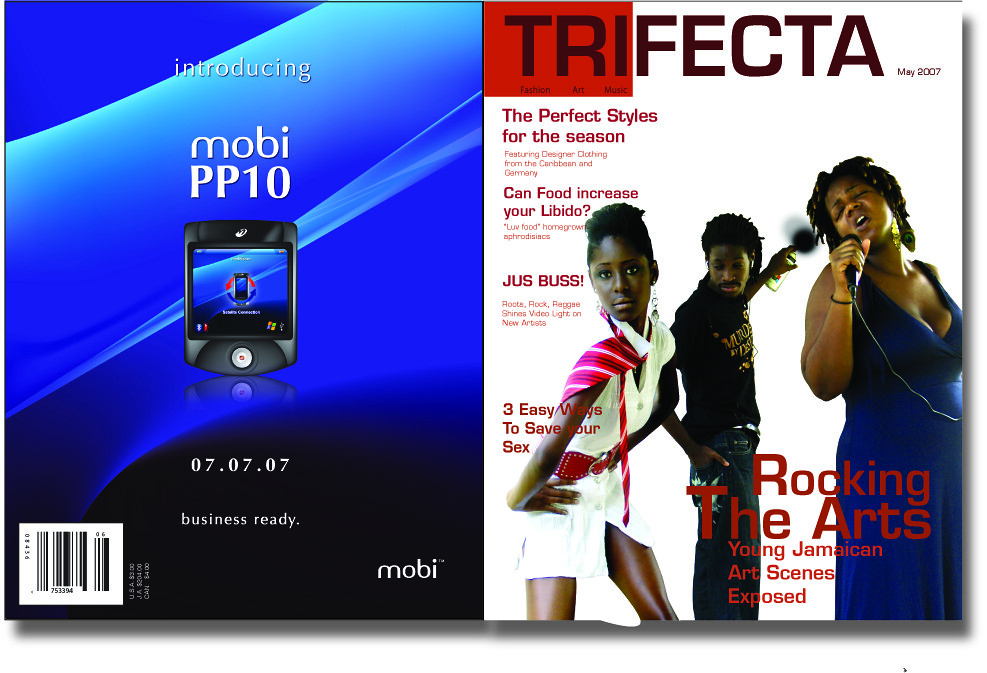This image shows both the front and back covers of a magazine titled "Trifecta," dated May 2007, laid flat. The front cover features vibrant and dynamic text along with three black individuals, presumably Jamaican, each in their late 20s. The headline articles include "The Perfect Styles for the Season," "Can Food Increase Your Libido?", "Three Easy Ways to Save Your Sex Life," and "Rocking the Arts: Young Jamaican Art Scenes Exposed." 

On the right side of the cover, a woman with dreadlocks, dressed in a blue dress, passionately sings with her eyes closed while holding a microphone in her right hand. At the center, a man with dreadlocks stands confidently in a black t-shirt with yellow writing and dark jeans, holding a spray paint can in his left hand, his arm slightly raised. To the left, another woman strikes a pose wearing a stylish white and red dress with a red belt and long earrings. 

The back cover on the left side features an ad for the Moby PP10 handheld device. The advertisement, set against a blue background, reads "Introducing Moby PP10," followed by the date "07.07.07" and the tagline "Business Ready." At the bottom, the Moby logo is positioned on the right, with a barcode on the left.